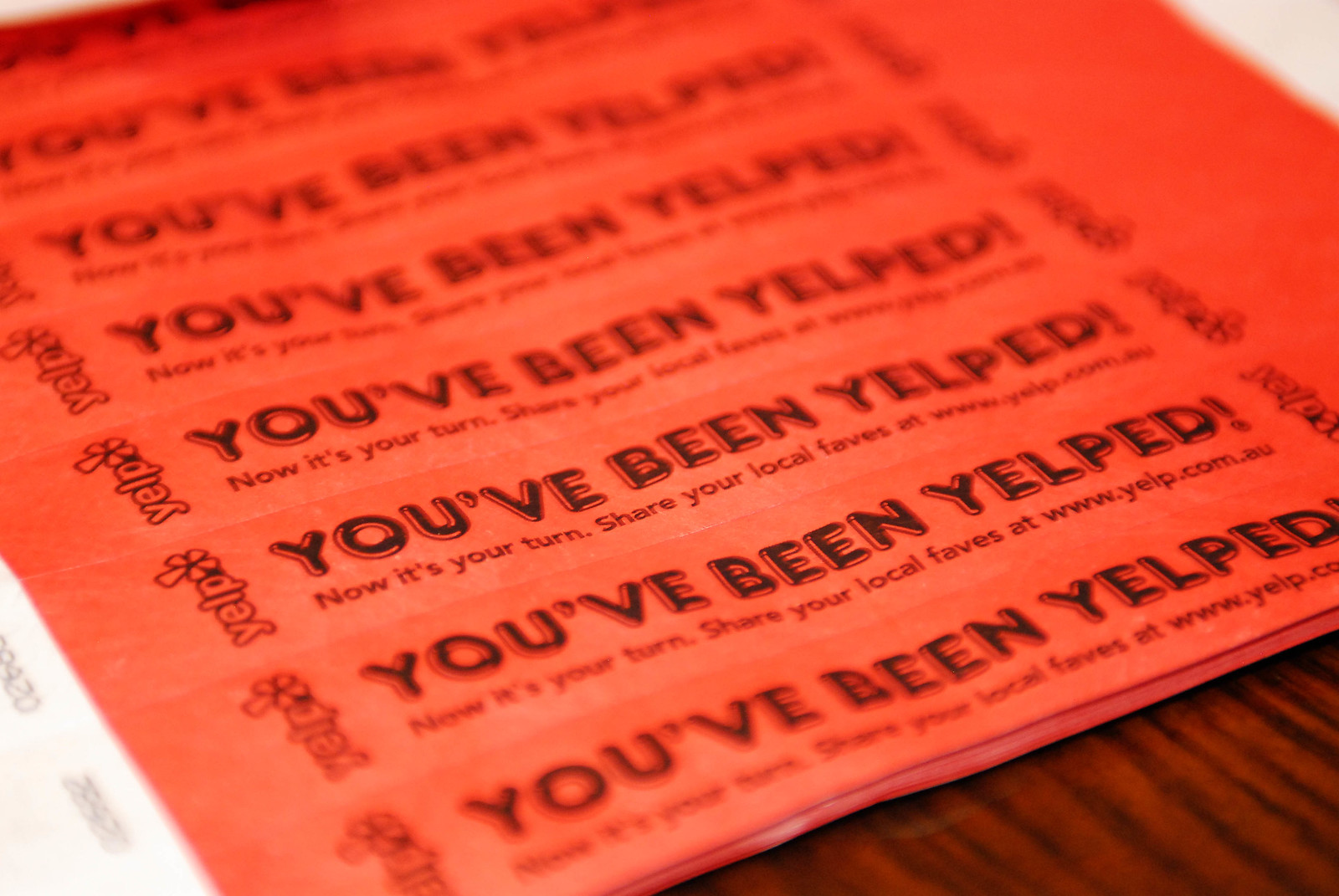In the image, we see a sheet of orange, perforated, wristband-like tags arranged diagonally across a dark reddish-brown wood grain table. The tags prominently feature the phrase "You've Been Yelped!" in uppercase, black bubble letters outlined in red, with an exclamation mark. Below this, it reads, "Now It's Your Turn. Share Your Local Faves at www.yelp.com." The slogan is repeated on each perforated strip, which can be easily torn off and shared. The Yelp logo is displayed sideways along both the left and right edges of the tags, albeit slightly blurred on the right side. There's a white strip on the left side, possibly for adhesive purposes. The table surface, rich in texture, adds a contrasting background to the vibrant orange tags.